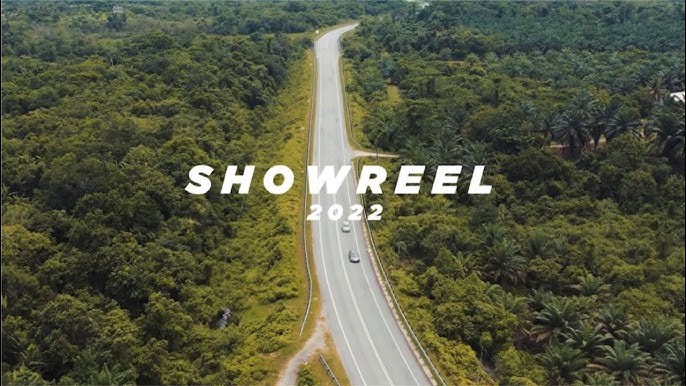This horizontal rectangular aerial photograph prominently features a highway cutting through a densely wooded area. The highway, consisting of two lanes in each direction, runs from the center bottom of the image to the top, where it curves to the right and vanishes behind a canopy of lush trees. Displayed in large white letters at the center of the image is "SHOWREEL 2022," marking the photograph as a visual highlight. On either side of the highway, the forest appears dense, filled with green, yellow, and brown leaves, creating a fluffy, dark-greenish texture from above. The left side of the frame is dominated entirely by this dense forest with no visible structures, while the right side includes a hint of a building near the far edge and a small dirt road leading to it, suggesting the presence of a farm. A minor path veers off to the left near the bottom of the image. A couple of cars are visible on the road, emphasizing the image's daytime brightness and the vivid natural surroundings.